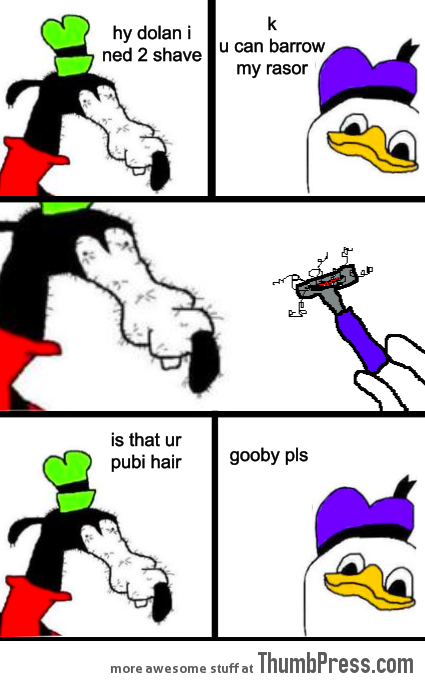The comic strip consists of five panels arranged horizontally in three sections, set against a white background. The top section features two panels. On the left, there's a caricature of Disney's Goofy, with exaggerated features including a green leprechaun hat, red shirt, and a distorted face devoid of eyes, displaying his teeth and black nose prominently. Goofy is depicted saying, “Hy Dolan, I ned 2 shave.” To the right, the second panel showcases a peculiar version of Donald Duck with a purple hat and a smirky expression, replying, “K, U can barrow my razer.”

The middle section contains a single cohesive panel showing Goofy's reaction and Donald's hand extending a razor. The razor, noticeably outlined in purple, is cluttered with hair.

The bottom section splits into two panels. On the left, Goofy questions, “Is that your puby hair?” with an emphasized misspelling. The right panel has a weary-looking Donald Duck responding with, “Gooby pls.” Beneath these panels, a small text caption promotes, “More awesome stuff at thumbpress.com.”